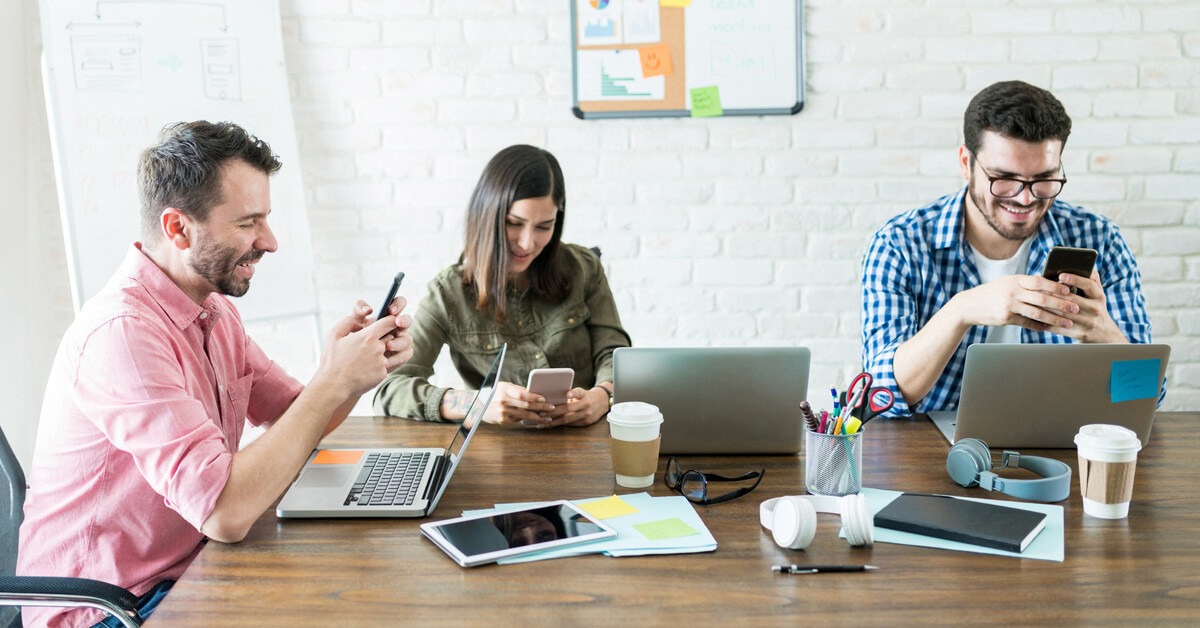In this image, three individuals are seated at a long, dark wooden conference table within a casual office setting characterized by white brick walls adorned with various bulletin and whiteboards. The table is cluttered with typical office items such as laptops, coffee cups, iPads, folders, papers, and a jar filled with pens and scissors, indicative of a meeting environment. All three individuals are engrossed in their cell phones.

On the far left is a man with short black hair, a neatly trimmed beard, and mustache. He is wearing a salmon-colored long-sleeve button-up shirt and smiling as he texts on his phone. Next to him is a woman with long brown hair, dressed in an olive green button-up shirt, also focused on her phone. To her right is another man in a blue and white plaid shirt over a white undershirt. He has a beard, black glasses, and short black hair and is intently using his phone as well. Each individual has a silver laptop in front of them, contributing to the busy, multi-tasking atmosphere of the setting. The background bulletin and whiteboards feature graphs, sticky notes, and various pieces of information, enhancing the professional context of the scene.